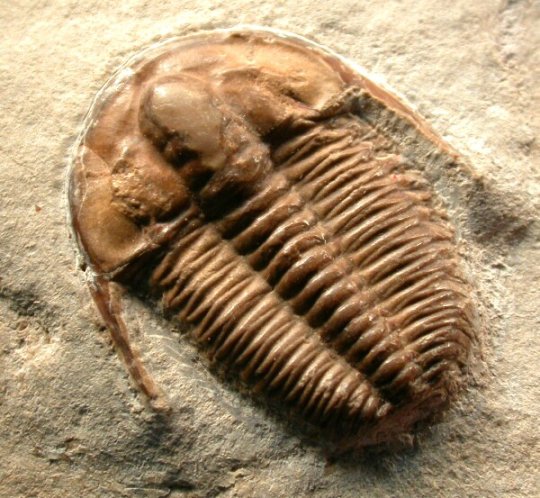The image portrays a well-preserved fossilized creature encased in rock, displaying a resemblance to a horseshoe crab, albeit with distinct differences. The fossil, which appears to be set in a rock matrix of gray, pink, and white hues, is primarily brown with gold and tan accents and possesses a somewhat shiny surface. The top part of the fossil features a smooth shell-like structure, while the central area showcases a ridged, spiny section leading into a textured lower portion adorned with lines. Notably, a line extends from the shell on the left side, further embedding into the surrounding rock. This undersea or perhaps even land-sea creature is reminiscent of a prehistoric species, and its alien-like appearance, especially with the spindly appendages, adds to its enigmatic nature. The fossil's intricate details and unique features hint at its possible scientific importance, suggesting it might be a specific yet unidentified ancient organism.